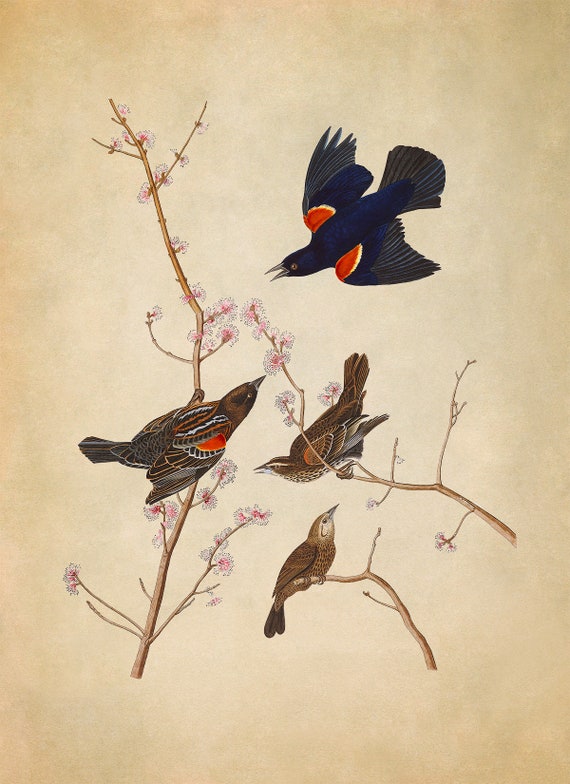This painting depicts an elegant scene of four birds set against an off-white, slightly darkened at the edges, creamy background, resembling old paper. Delicate light pink cherry blossoms with thin, floating stems embellish the composition. At the bottom left, a brown bird with a touch of red on its wings gazes upward. To its right, another brown bird with subtle orange wing markings looks towards a fellow bird. Above these two, perched on branches with no leaves and just light pink and white flowers, is a brown bird seemingly observing its companions. Gracefully flying overhead, a red-winged blackbird with a pointed beak, yellow eyes, and wings spread wide adds a sense of movement, swooping down from the top right corner. The detailed juxtaposition of the vivid bird colors and the subtle blossoms creates an air of refined elegance throughout the artwork.